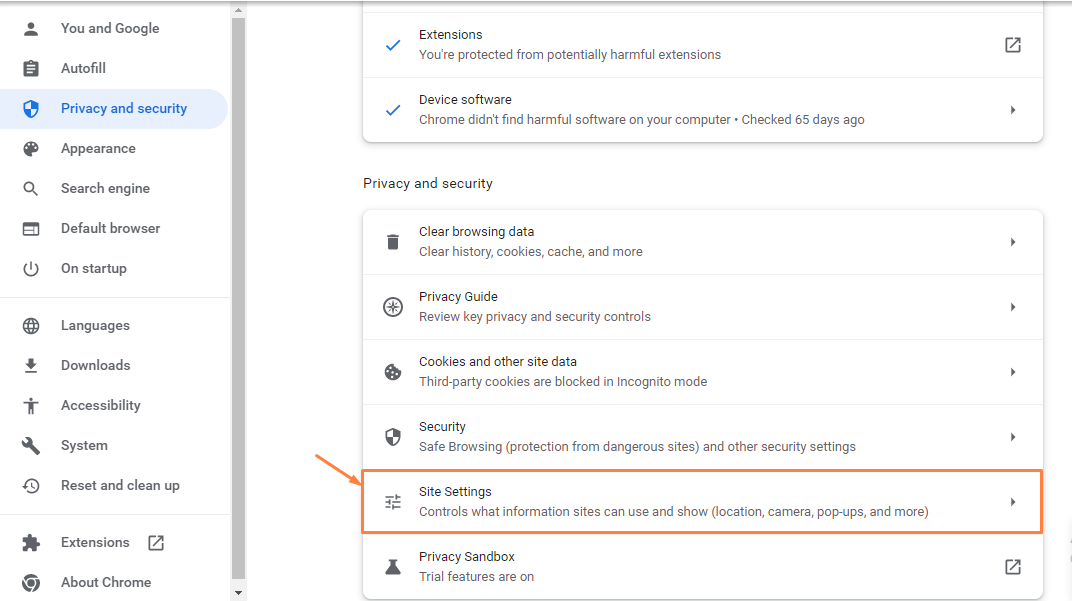The image depicts a user navigating their settings on a website. The interface has a thin gray border at the top and a wider gray border starting at the top-left portion of the screen. The background is white with margins approximately two inches from the left. 

On the left side, a column of icons is displayed, each representing a different settings category. To the right of this column, there are corresponding descriptions of each icon. The first icon represents a profile with the label "You and Google" in black text. The second icon represents autofill settings, simply labeled "Autofill." The third icon is a shield, indicating "Privacy and Security," highlighted in blue with a light blue border around it.

Beneath these, the settings categories continue with: 
- Appearance
- Search Engine
- Default Browser
- On Startup
- Languages
- Downloads
- Accessibility
- System
- Reset and Cleanup
- Extensions 

Each category has a unique icon beside it.

On the right side of the screen, a small rectangle presents options with blue checkmarks on the left. The first option is labeled "Extensions," followed by a description. Underneath that, "Device Software" is detailed with information on the last check, marked by a line. The top rectangular option features an upward-pointing arrow, while the second has a gray band sign pointing to the right.

Further down, in a labeled space, "Privacy and Security" is prominently displayed in black text. Below this, the icons on the left are accompanied by their corresponding descriptions and additional information on the right. The fifth icon down is highlighted with an orange rectangle, featuring a downward and rightward-pointing arrow beside it, designated for "Site Settings." This icon is placed below four other icons.